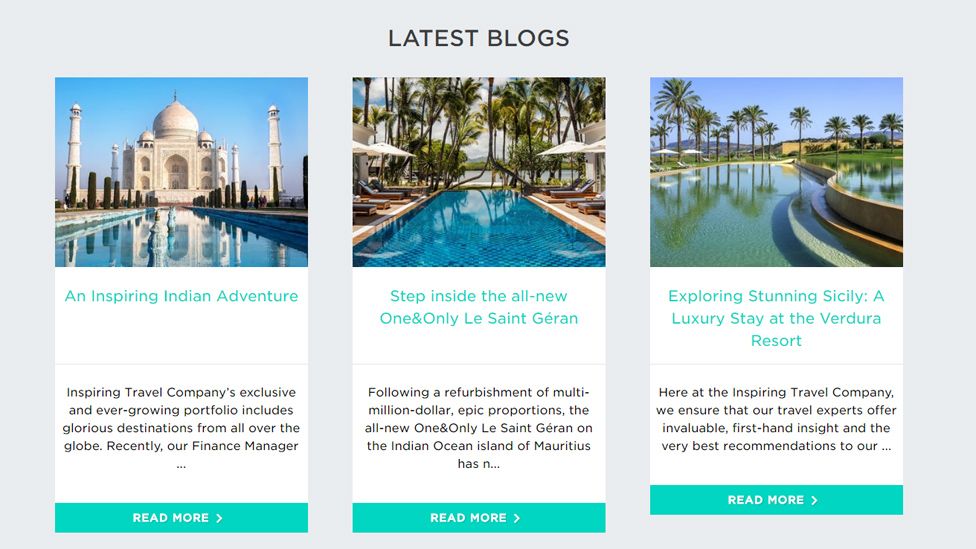In this visually appealing image, the heading "Latest Blogs" is prominently displayed at the top against a light grayish blue background in bold black text. Below the heading, three captivating photographs are aligned horizontally, each accompanied by descriptive text and a "Read More" call to action.

1. **Left Photograph**: Features the iconic Taj Mahal under a clear, cloudless blue sky, with its majestic reflection shimmering in the pool in the foreground. The text below reads in blue, "An Inspiring Indian Adventure." A horizontal line divides this from the additional text, which states in black, "Inspiring Travel Company's Exclusive and Ever-Growing Portfolio Includes Glorious Destinations from All Over the Globe. Recently, our Finance Manager..." A teal bar at the bottom has "Read More" in white, accompanied by a rightward arrow.

2. **Middle Photograph**: Depicts a serene swimming pool surrounded by lush palm trees and inviting lounge chairs. Below this, blue text reads, "Step Inside the All-New One and Only Le Saint Juran." Another horizontal line separates this from the accompanying text, which says in black, "Following a Refurbishment of Multi-Million Dollar Epic Proportions, the All-New One and Only Le Saint Juran on the Indian Ocean Island of Mauritius has n..." The bottom teal bar features "Read More" in gray text with a rightward arrow.

3. **Right Photograph**: Shows a luxurious scene that includes a swimming pool bordered by palm trees, loungers with white umbrellas, and a clear blue sky. Below, the light blue text reads, "Exploring Stunning Sicily, a Luxury Stay at the Verdura Resort." A horizontal line divides this from the following black text, "Here at the Inspiring Travel Company, we ensure that our travel experts offer invaluable first-hand insight and the very best recommendations to our..." At the bottom, a teal banner has "Read More" in gray letters with a rightward arrow.

This detailed and descriptive layout showcases the alluring attractions and luxurious travel experiences presented by the Inspiring Travel Company, inviting readers to explore further by clicking on the "Read More" links.